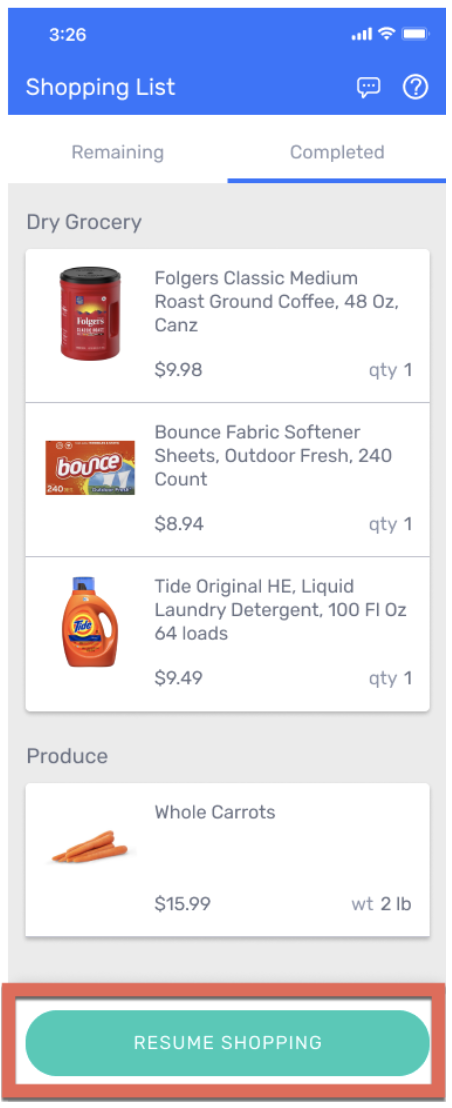This vertically-oriented image depicts a mobile device screenshot captured at 3:26 PM with the battery almost fully charged, as indicated by the blue bar at the top. Below the blue bar, the header reads "Shopping List" in white text. Underneath the header is a smaller white bar with two options: "Remaining" on the left and "Complete" on the right. The "Complete" option is selected, denoted by the blue line underneath it.

The rest of the screenshot features a gray background and lists a few products under the heading "Dry Grocery." The products are displayed in horizontal white boxes, each containing a product image, name, description, and price. 

1. The first product is "Folgers Classic Medium Roast Ground Coffee, 48 ounces" priced at $9.98. The image shows a red can with a black cap.
2. The second product is "Bounce Fabric Softener Sheets, Outdoor Fresh, 240 count" priced at $8.94. The image depicts an orange box with white sheets hanging outside against a blue sky.
3. The third product is "Tide Original HE Liquid Laundry Detergent, 100 fluid ounces, 64 loads" priced at $9.49. The image shows an orange Tide jug.

At the bottom of the screenshot, there's an entry for "Whole Carrots" accompanied by a picture of carrots.